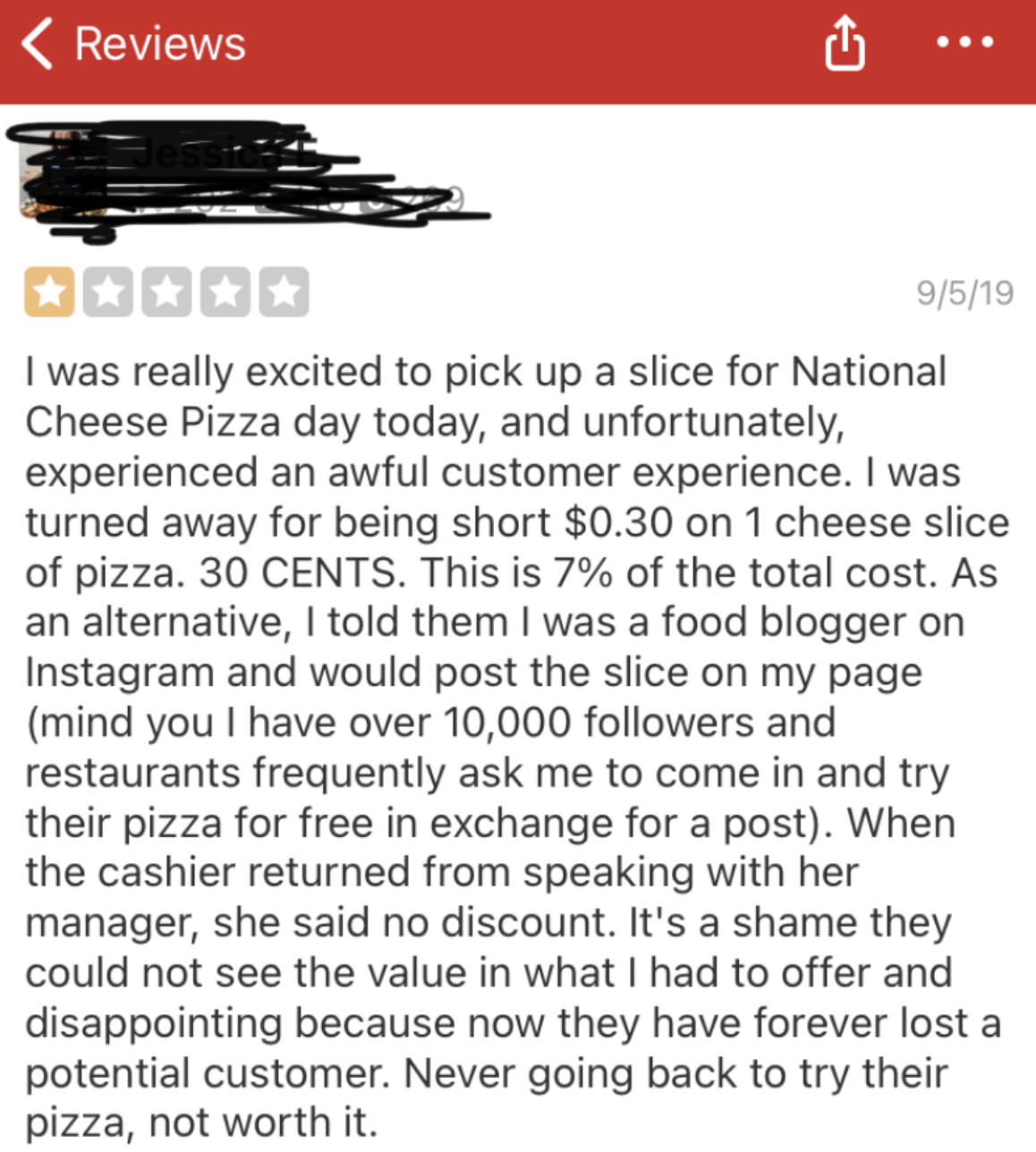The image depicts a review with the following elements:

- **Top Section:** The top inch of the image features a dingy red color in the top left corner. There is a prominent white "greater than" sign pointing left, followed by the word "Reviews" in white text. On the upper right side, there are three white dots and a white download icon.

- **Reviewer’s Information:** On the left side, the reviewer's name has been blacked out. Directly below this, there is a rating indicator showing one yellow square with a white star, followed by four gray squares with gray stars, indicating a one-star rating. On the far right, the date "9/5/19" is displayed in black text.

- **Review Content:** The main body of the review is a lengthy paragraph detailing a negative experience:
  - The reviewer was excited to purchase a slice of cheese pizza for National Cheese Pizza Day.
  - They were turned away for being 30 cents short on one slice of pizza, which amounted to 7% of the total cost.
  - As an alternative, the reviewer mentioned being a food blogger on Instagram with over 10,000 followers and offered to post about the slice in exchange for it.
  - After the cashier consulted with the manager, they were denied any discount.
  - The reviewer expressed disappointment that the establishment could not see the value in their offer and stated they would never return, deeming the pizza unworthy.

This review highlights the customer's frustration and the lost opportunity for the restaurant to engage with a potentially influential social media presence.